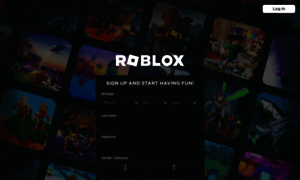The image depicts the login screen of Roblox. Dominating the center is the prominent "Roblox" logo in white text. Below the logo, there is a black pop-up square that contains the prompt, "Sign up and start having fun," with fields for inputting user information. In the top right corner, there is a white rectangular button labeled "Login."

The background is a mosaic of various vibrant scenes from Roblox, featuring different colors and elements of the game, arranged in a series of squares. These squares are set at a diagonal tilt, creating a dynamic visual effect. Three full rows of these squares are visible, with partial rows peeking from the top right and bottom left corners. The squares are separated by sleek black lines that add definition to the background. The overall layout and colorful imagery capture the diverse and engaging nature of Roblox.